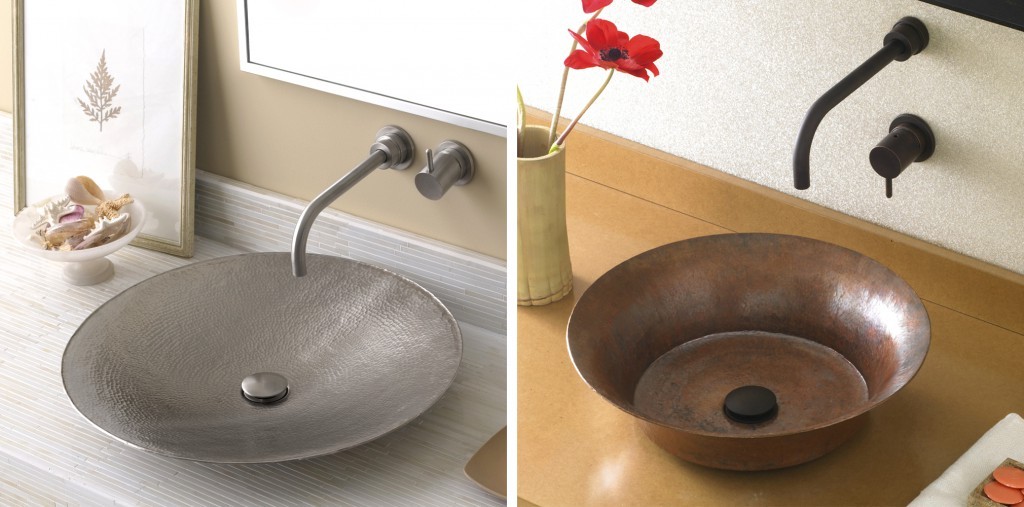The image depicts two distinct sink setups, each showcasing unique design features. The left sink features a shallow, saucer-like silver bowl with a matching silver faucet and handle built into the tan-colored wall. Above the sink, there's a white-framed mirror and to the left, a white bowl filled with various seashells sits on the gray wooden counter. Behind the seashell bowl, there's a picture frame displaying a plant against a brown background. The right sink, in contrast, utilizes a deeper bronze bowl positioned on a similar light gray wooden surface. The bronze faucet and knob are also mounted on the wall, maintaining a cohesive design theme. Both setups exhibit their own distinct style, with the left emphasizing clean, modern lines and the right integrating deeper, more rustic elements.